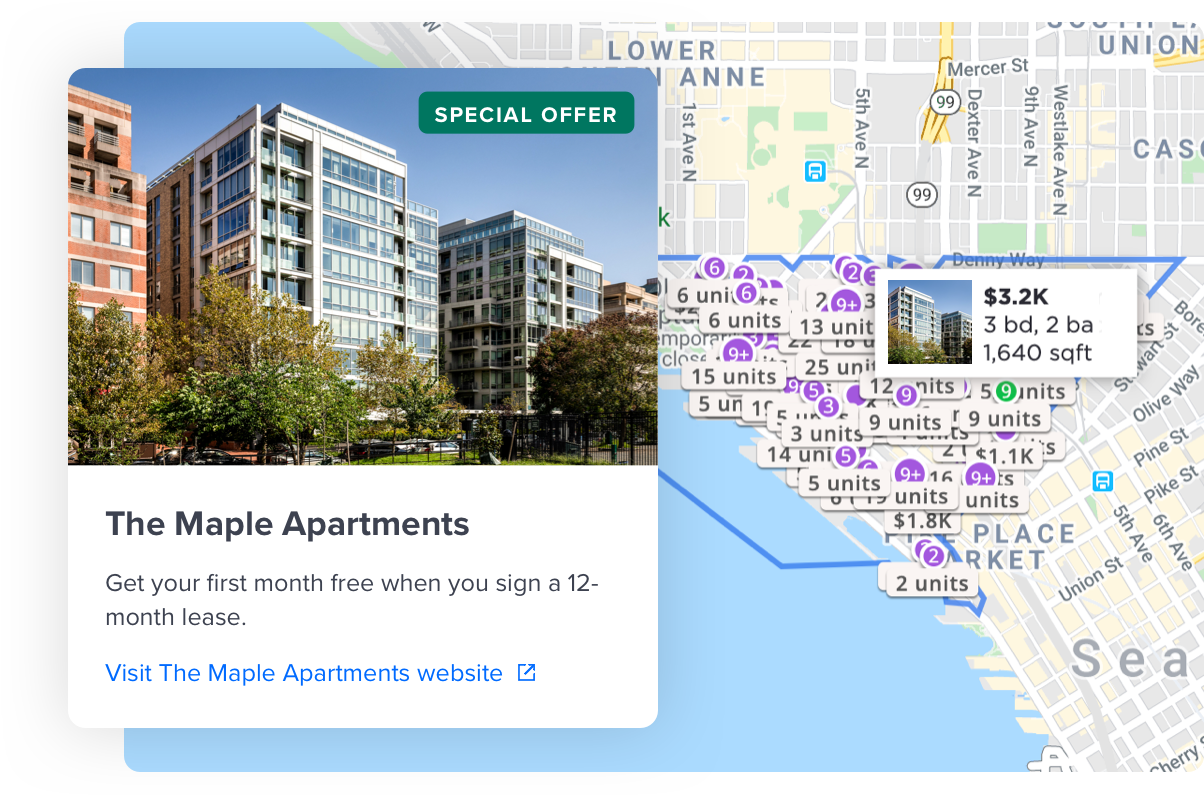The image is a detailed screenshot of an interactive map showcasing various housing options available for rent in downtown Seattle, specifically around the Pike Place Market area. On the left side of the image, there's a prominent picture of apartment buildings with a green banner overlay that reads "Special Offer" in white font. Below this banner, the text "The Maple Apartments" is displayed, accompanied by a promotional offer: "Get your first month free when you sign a 12-month lease." Additionally, a blue link urges viewers to "Visit the Maple Apartments website."

The map, which serves as the background, is filled with various icons indicating the availability of units in different buildings—such as "3 units," "9 units," "5 units," and "15 units." The specific listing highlighted prominently in the image indicates a rental price of $3.2k per month for a 3-bedroom, 2-bath apartment with a spacious area of 1,640 square feet.